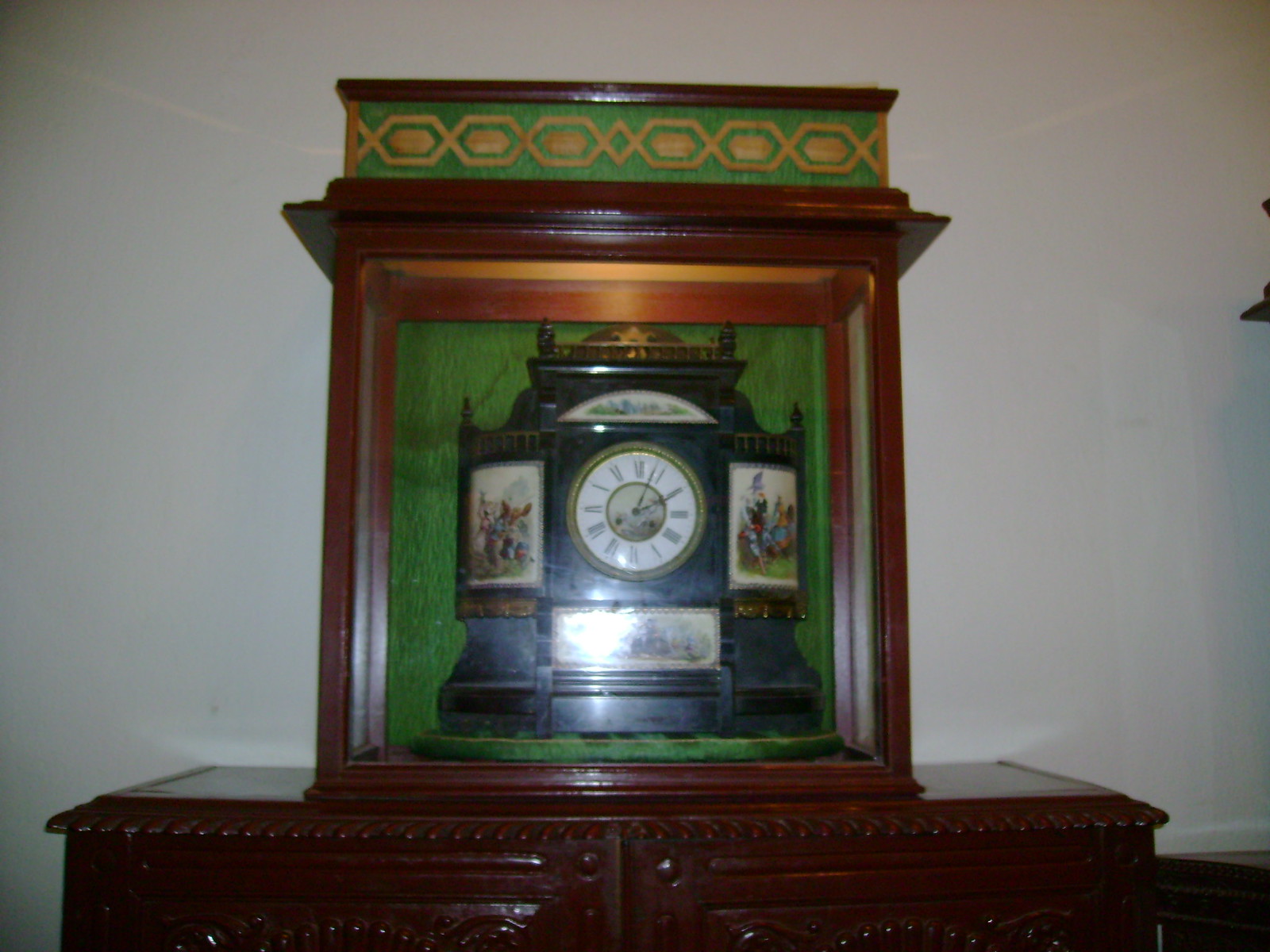The photograph showcases a very ornate clock encased in glass, perched atop an elaborately carved, dark wooden chest of drawers with a reddish tint. The dresser features several drawers and decorative trim. The display case containing the clock has a wooden frame and is capped with a green and gold inlaid pattern, resembling felt or a cloth material with a hexagonal design in the center. The clock itself, almost black in color, has an ornamental design with multiple faceted sides and white porcelain inlays. The clock face is white with Roman numerals, surrounded by a gold trim both on the outer edge and in the center where the hands are located. This center section also features a detailed drawing. At the top of the clock, there are finials and spires, with a crescent moon-shaped porcelain piece. Above and below the clock are paintings, and there's an unreadable white plaque beneath it due to a reflective light. The intricate design and exotic elements suggest a possible Southeast Asian influence, making it a truly captivating piece.